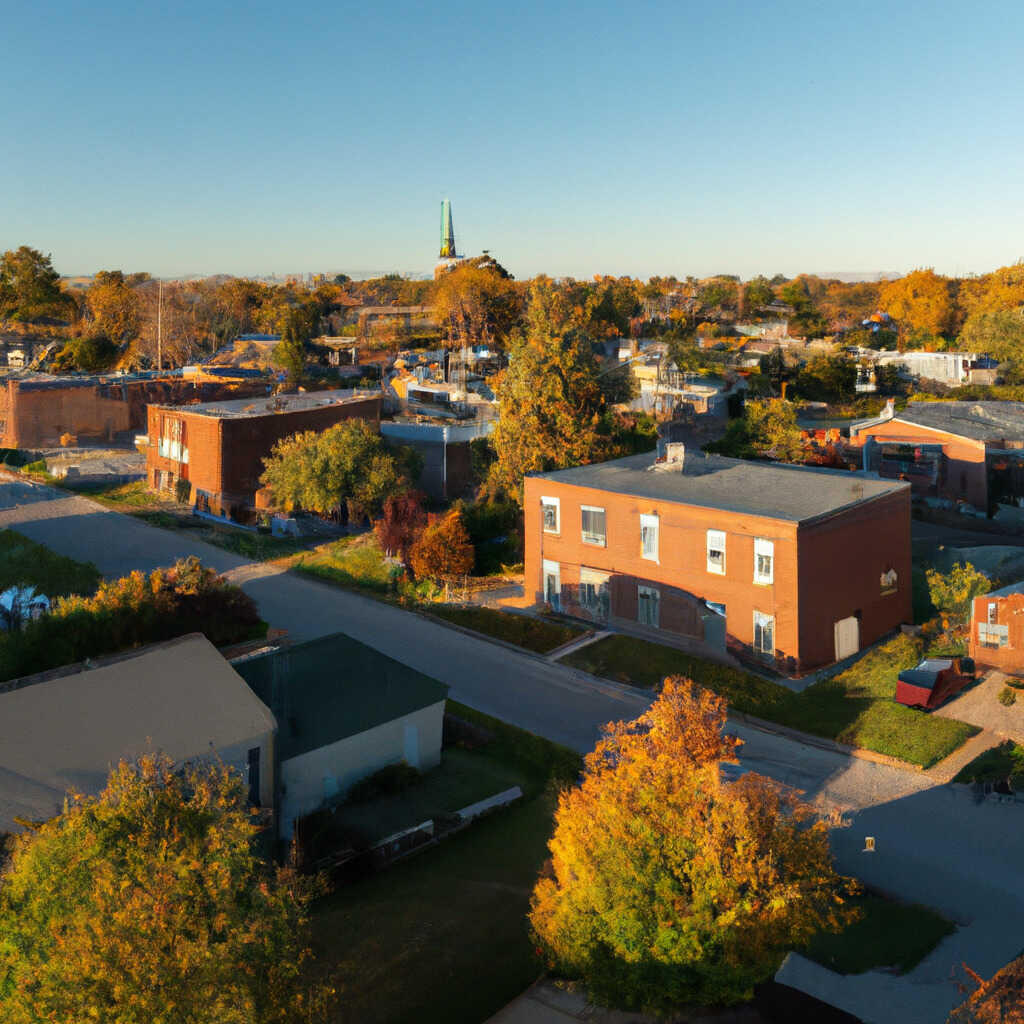The photograph depicts a suburban scene from a slightly elevated bird's-eye view, focusing on a street lined with numerous small buildings. The scene is characterized by an abundance of trees, showcasing a mix of vibrant greens and autumnal oranges, indicating the transition into fall. The buildings, primarily constructed from red and brown brick, appear to be in various states of disrepair. Despite their small size, they resemble compact residential units rather than large apartment complexes or businesses. One prominently centered building features ten windows and a possible door on the ground level, with a trash can visible out front. Driveways can be seen leading up to these buildings, which are scattered across lush, green lawns. 

In the far background, a tall spire is visible, likely belonging to a church, along with a possible factory exhaust pipe. A horizontal strip of blue sky traces the top of the image, enhancing the expansive feel. The roadway, intersecting the scene from the left-hand side to the bottom right-hand corner, is flanked by grassy areas, including a gray house with an attached garage in the lower left corner. Small vehicles are sporadically placed along the street, adding to the suburban atmosphere.